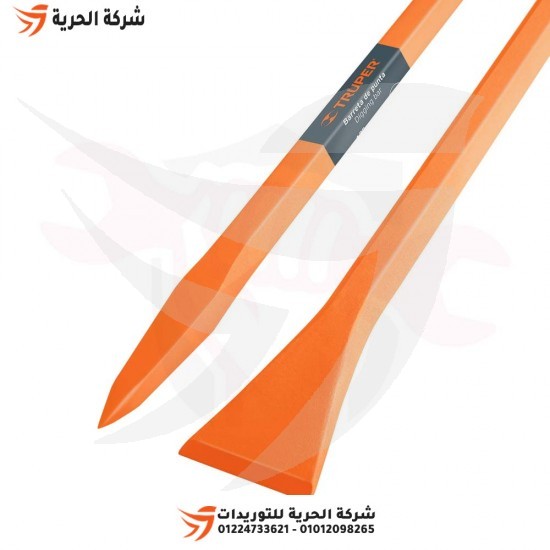This is an image of an advertisement for tools featuring two thin, orange items positioned diagonally side-by-side in the center against a white background. The top item has a pointed bottom and a black tape-like label that reads "Audit Trooper," spelled T-R-U-P-E-R. Below that, it indicates "Beretta de Puente Digging Bar." The bottom item is flat, resembling a scraper. Both items are thin and handle-like in appearance. A logo and Chinese lettering are present in the top left corner, with the same symbol, Chinese characters, and product codes including "01224733621-012247" and "0101209-8265" repeated at the bottom. Gray images of Japanese or Chinese symbols appear throughout the background as a watermark.